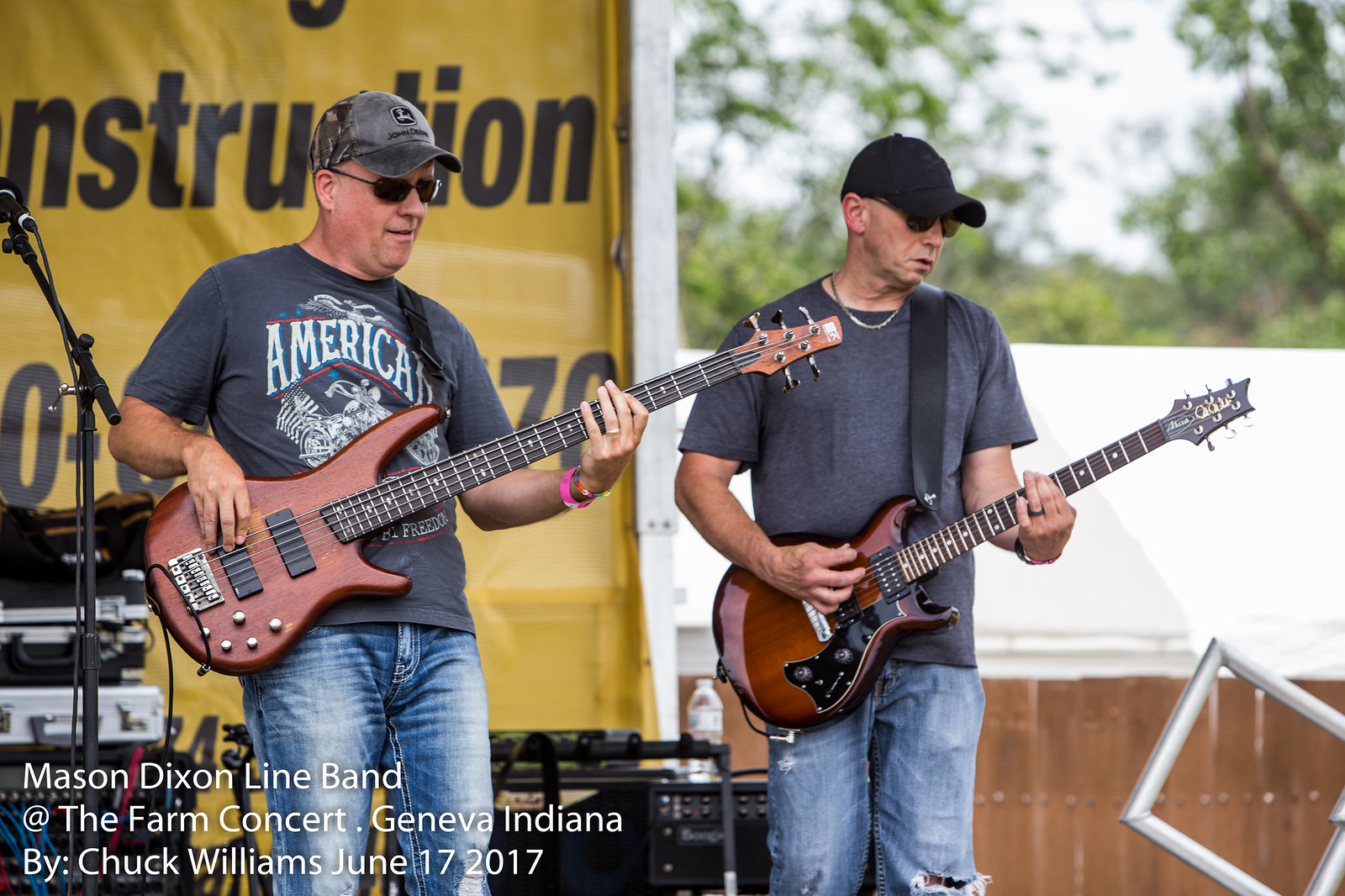In this horizontally oriented photograph of the Mason Dixon Line Band performing at the Farm Concert in Geneva, Indiana on June 17, 2017, captured by Chuck Williams, two male guitar players are featured on stage. Both musicians are engrossed in their performance with electric guitars in hand. The musician on the left is wearing a gray John Deere camouflage cap, dark sunglasses, and a gray graphic T-shirt that says "America," paired with blue jeans. His guitar is a mahogany electric, and his playing style suggests he might be handling it like a bass guitar. The musician on the right dons a black baseball cap, sunglasses, a plain gray T-shirt, and blue jeans, and he is playing his electric guitar with a pick. Behind them, a yellow banner with black writing, reminiscent of a construction sign, serves as the backdrop. The stage is equipped with standard concert paraphernalia, including a microphone and a bottle of water. In the lower left-hand side of the photo, text reads "Mason Dixon Line Band at the Farm Concert, Geneva, Indiana, by Chuck Williams, June 17, 2017." The background also features a brown fence, an indistinct white roofline, some sort of glass object, and green foliage suggesting a summertime setting.